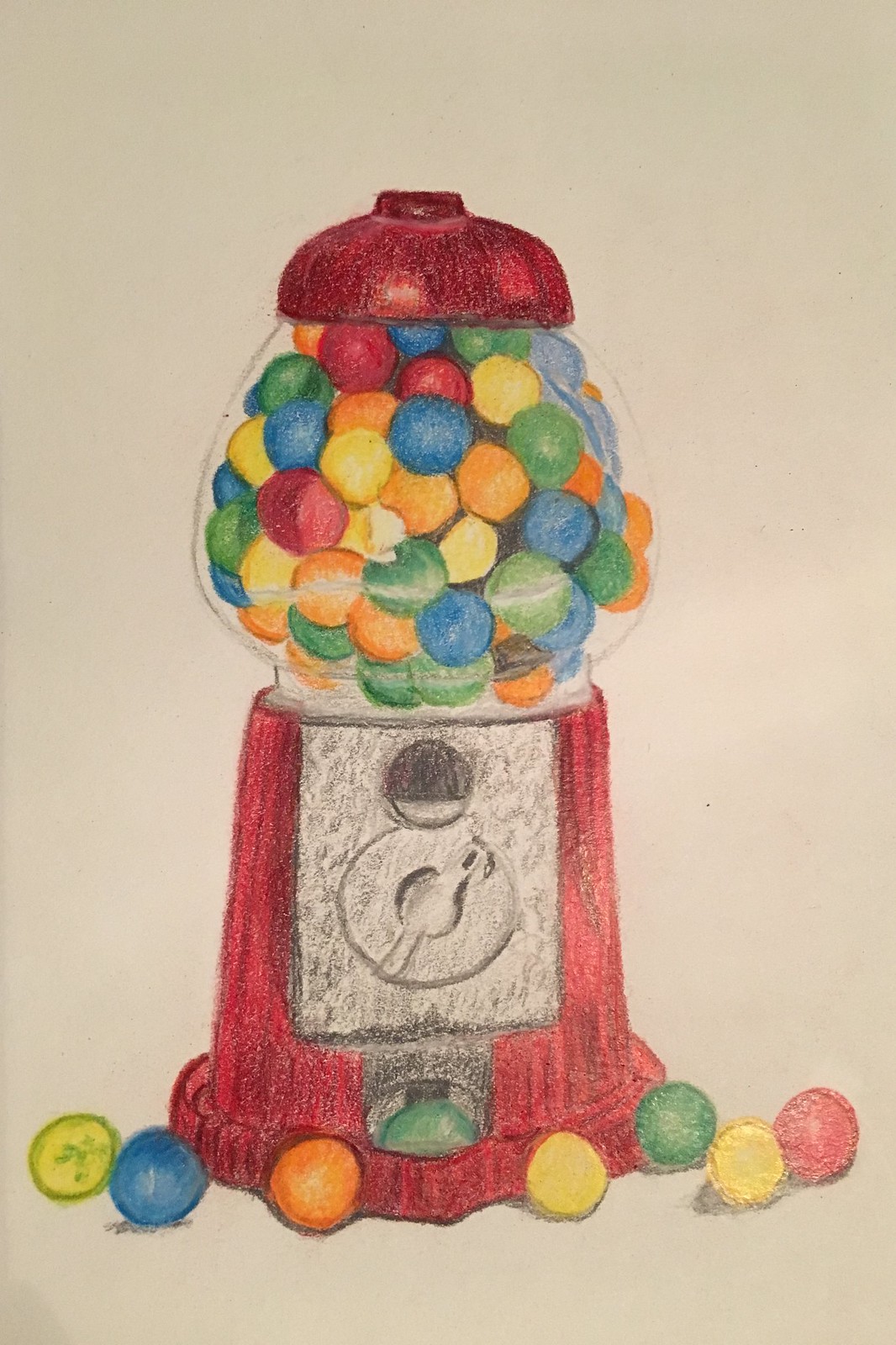In this detailed colored pencil drawing, a classic coin-operated gumball machine stands against a tan background, rendered with a vivid array of colors and realistic shading. The gumball machine features a red domed metal top and a clear, glass-like orb filled to the brim with gumballs in assorted hues of yellow, orange, red, blue, green, and light blue. This glass sphere captures the essence of translucence, showcasing the reflective properties of both the glass and the vibrant gumballs inside. 

The machine itself has a red metal base that tapers at the bottom, with a shiny silver section in the center that houses the coin slot and the dial for dispensing gumballs. The gumballs at the machine's base include a distinct pattern starting from left to right: a yellow, a blue, an orange, followed by another yellow, a green, another yellow, and then a red gumball. This artwork, likely executed with colored pencils on lighter cream or butcher block-colored paper, combines vibrant colors and intricate details to create a remarkably realistic and nostalgic piece.